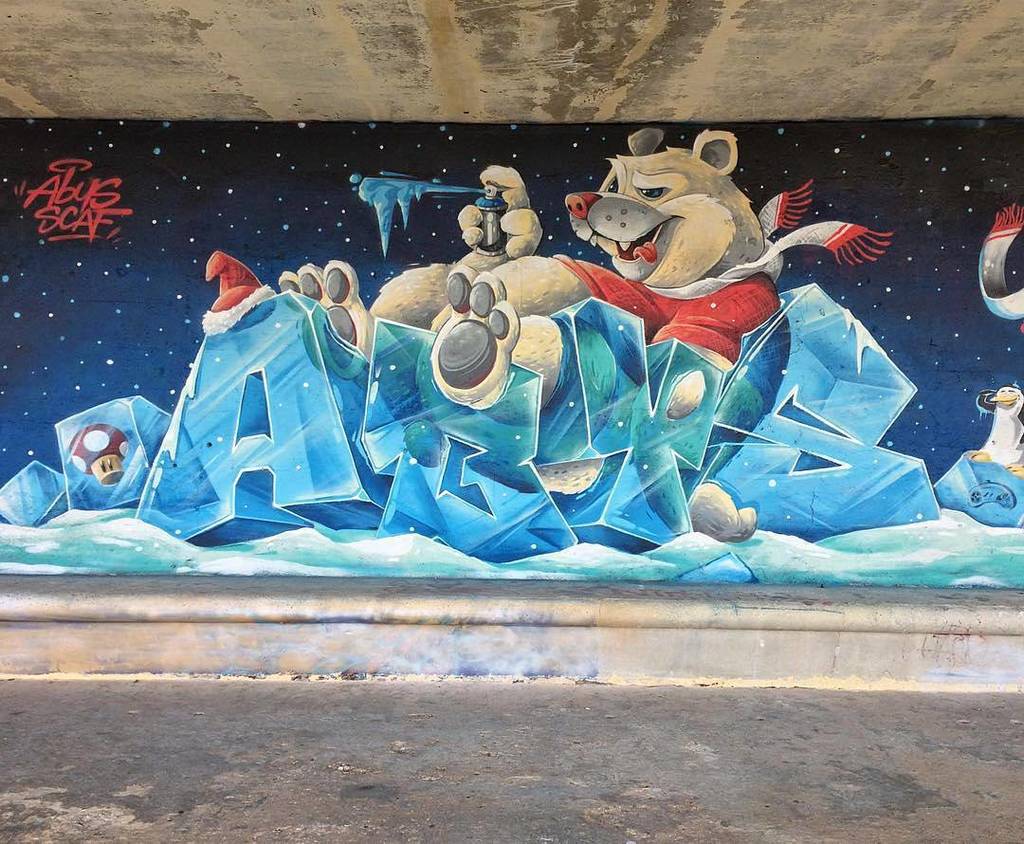The image is a detailed graffiti-style mural by an artist named Abus Scaf, situated beneath a bridge. It features a cartoonish polar bear as the central figure, positioned against a night sky backdrop adorned with blue hues and white stars. The bear, dressed in a red shirt and a white-and-red scarf, has a distinctive red nose and is seen relaxing on top of large ice blocks that spell out "ABYS" in bold, icy letters. Above the letters, "SCAF" is written in red on the upper right side, adding a personal touch from the artist.

The bear's playful nature is highlighted by its tongue hanging out of the side of its mouth and it appears to be having fun spraying a can of paint, with vibrant blue splashes emanating from it. The spray paint also transforms into a large icicle. Additionally, a red-and-white Santa hat perches atop the letter "A" adding a festive flair, while other whimsical elements, such as a penguin sitting on an ice block designed as a game controller and a mushroom with eyes, are frozen beneath the ice. This mural combines intricate graffiti art with imaginative storytelling, creating an engaging and visually rich scene.